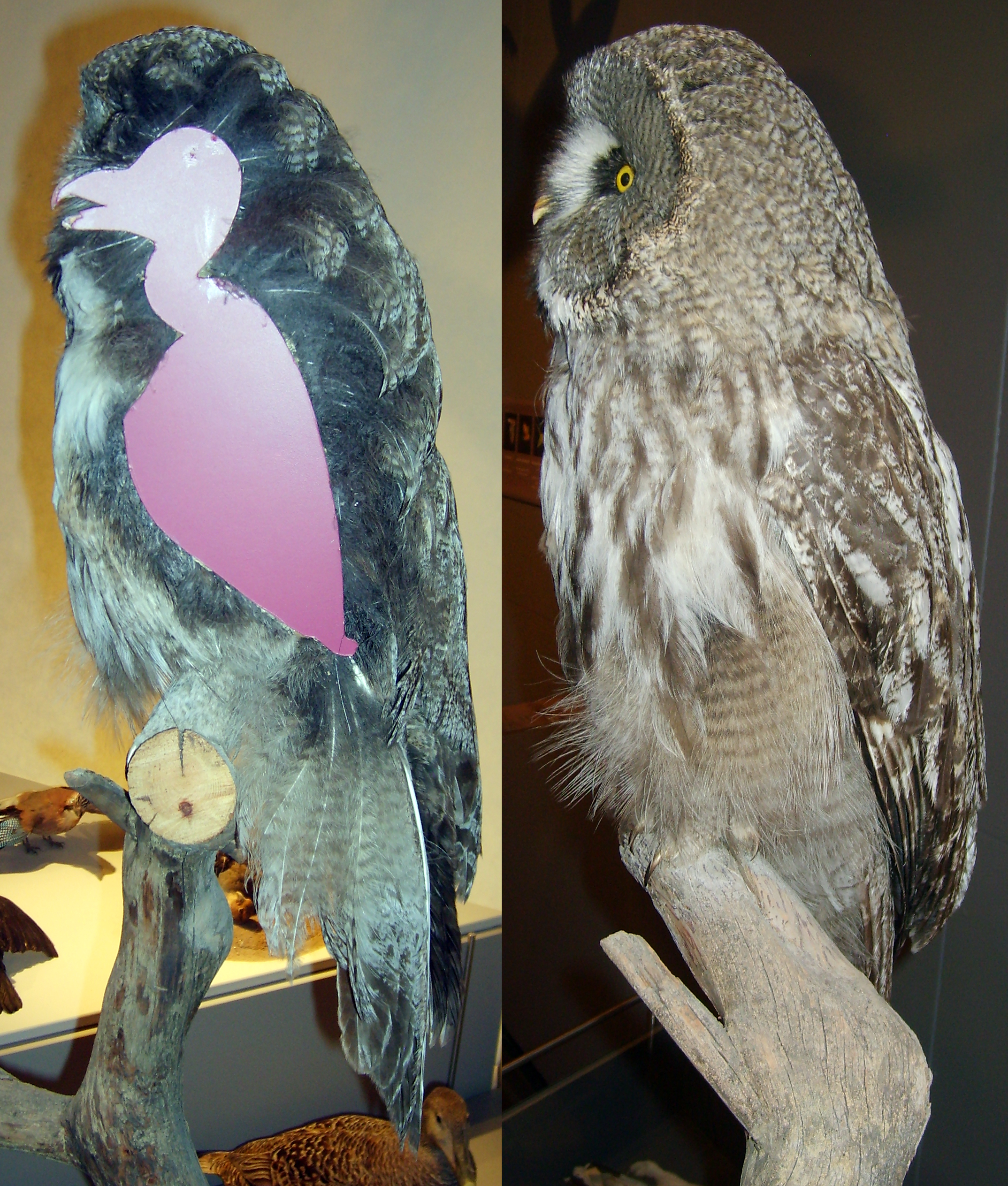The composition consists of two vertically split images juxtaposed against an off-white wall. On the right, a lifelike but still owl perches on a branch, its detailed feathers suggesting it might be a carefully crafted piece of taxidermy. The owl's plumage features a speckled pattern of white and brown on its chest and back, with a tan coloration towards the top. Its eyes are distinct with a yellow hue, adding a touch of realism that intimates taxidermy craftsmanship.

Contrasting this, the image on the left portrays another branch with the silhouette of an owl's body. However, the body is cut away to reveal a peculiar internal shape, which appears to be a pink representation reminiscent of a flamingo. This intriguing detail suggests a step in the taxidermy process or a conceptual art piece. At the bottom of this image, a duck can be seen, adding another layer of complexity to the visual narrative. Both images are unified by the plain off-white wall in the background, which serves to highlight the intricate details of the subjects.